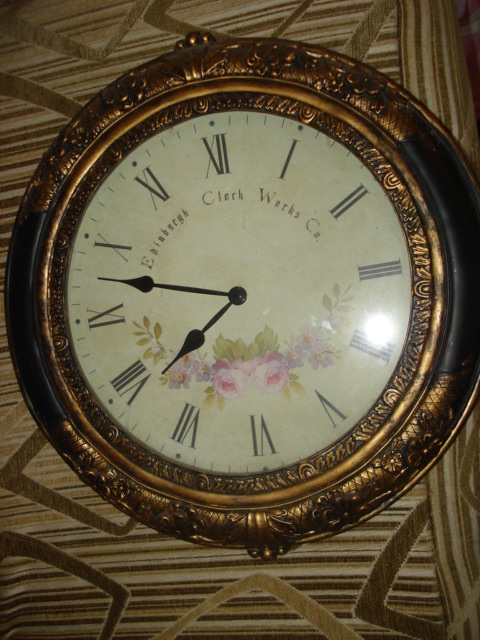This image captures a richly detailed Baroque-style clock, featuring an intricately designed frame that appears to be crafted from either copper or gold. The sides of the clock frame are darkened, resembling a soot-like color, which adds a dramatic contrast to the opulent metalwork. At the center, the clock face displays Roman numerals ranging from I to XII, accompanied by an hour and a minute hand, indicating the time as 9:39, though it's unclear if it is AM or PM. Inscribed on the clock face is "Edinburgh Clock Works Company," adding a touch of historical and locational context. The frame is embellished with a delicate floral design, enhancing the overall elegance and vintage charm of the timepiece.